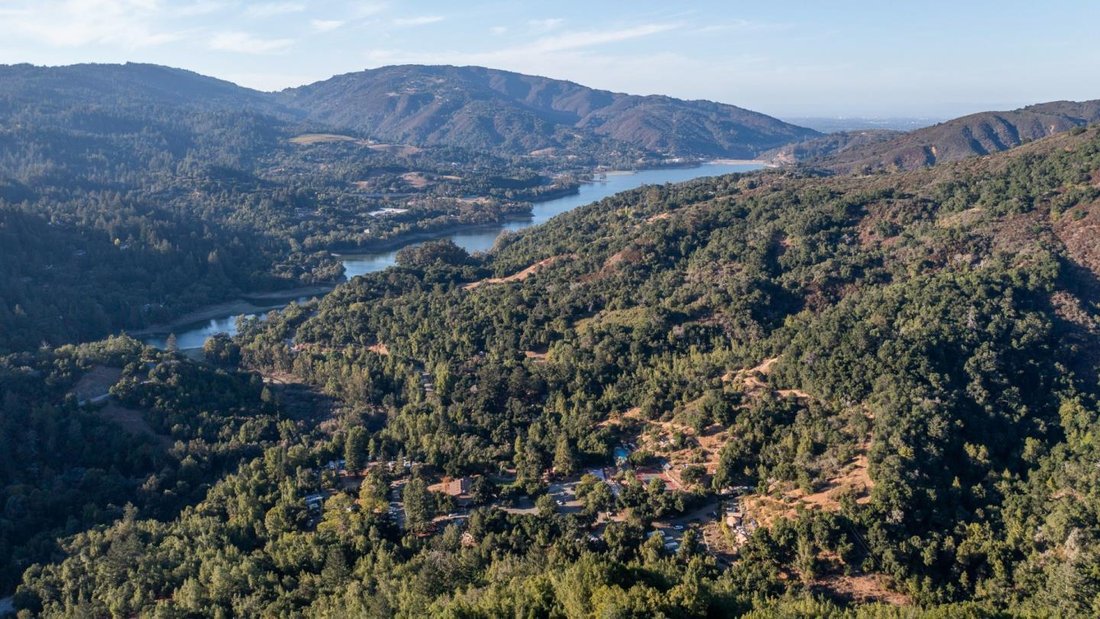This stunning aerial view, likely captured from an airplane or helicopter, showcases a lush valley with a winding river at the center. The scene is viewed from an angle, highlighting the varied landscape. At the top of the image, a light blue sky is punctuated with patches of white and gray clouds, overlaying a distant hilly skyline. The river begins at the top center, meandering down diagonally to the left before disappearing off the side of the frame. On the left side of the river, there is a gentle, grassy hill, while the right side features a rich, green valley densely populated with large trees intermixed with some brown patches, possibly indicating dirt paths or lighter foliage. Sparse buildings can be hinted at beneath the canopy of trees. The interplay of shadows, suggesting the soft light of early morning or late afternoon, casts dramatic reliefs on the landscape, particularly noticeable on the left side where the shadow deepens.